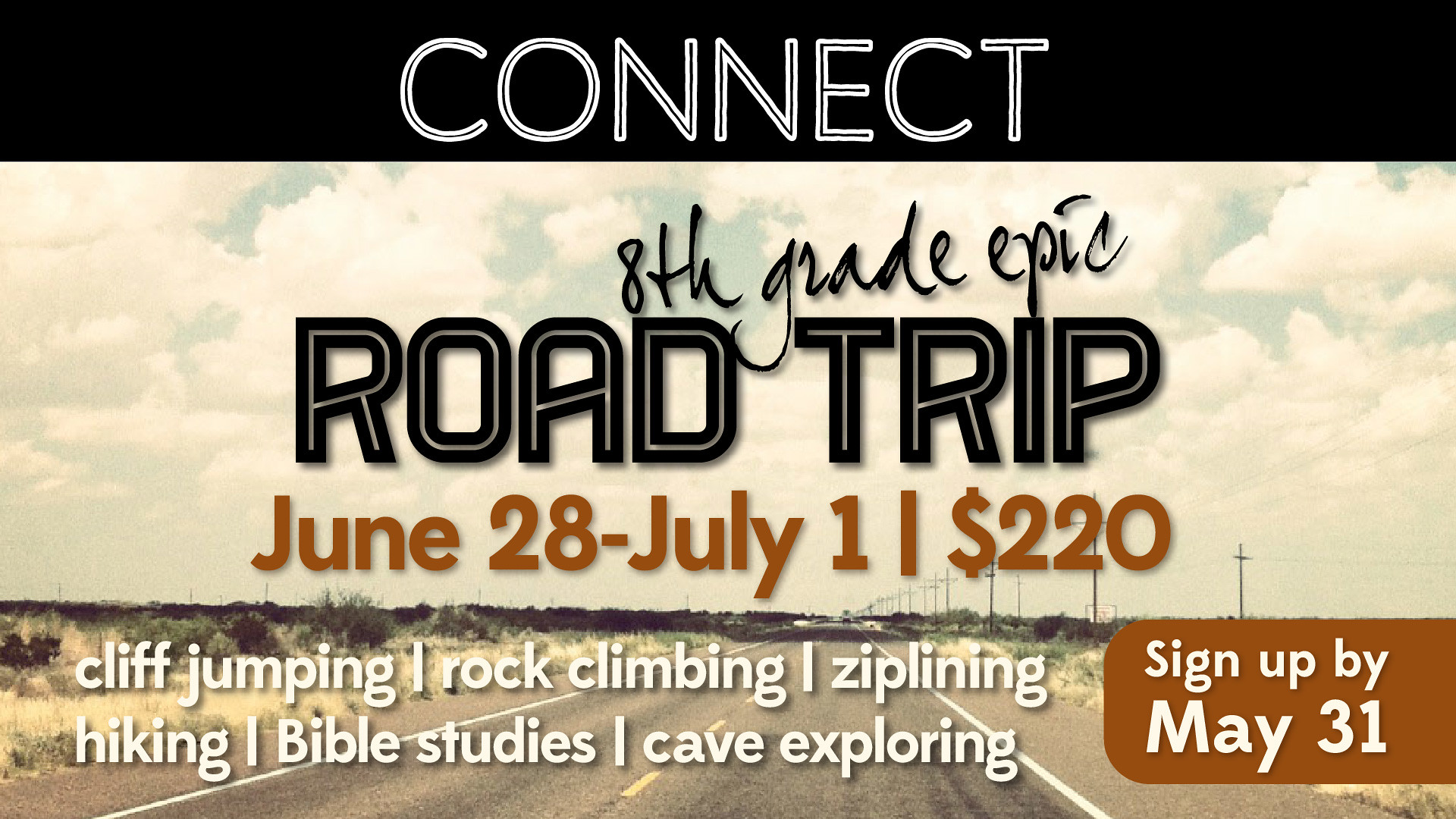This is an advertisement poster for an eighth-grade end-of-year epic road trip event. At the top, there's a black rectangle with bold, white, outlined text reading “CONNECT.” Below, a photograph features a straight desert road with sparse vegetation and power lines under a cloudy sky. Superimposed on the image, elegant script font announces “8th Grade Epic Road Trip,” followed by bold, black-outlined dates "June 28th - July 1st" and the cost "$220" in orange font. Beneath these, white text lists activities: cliff jumping, rock climbing, zip lining, hiking, Bible studies, and cave exploring. On the bottom right, an orange section with white text urges, “Sign up by May 31st.”